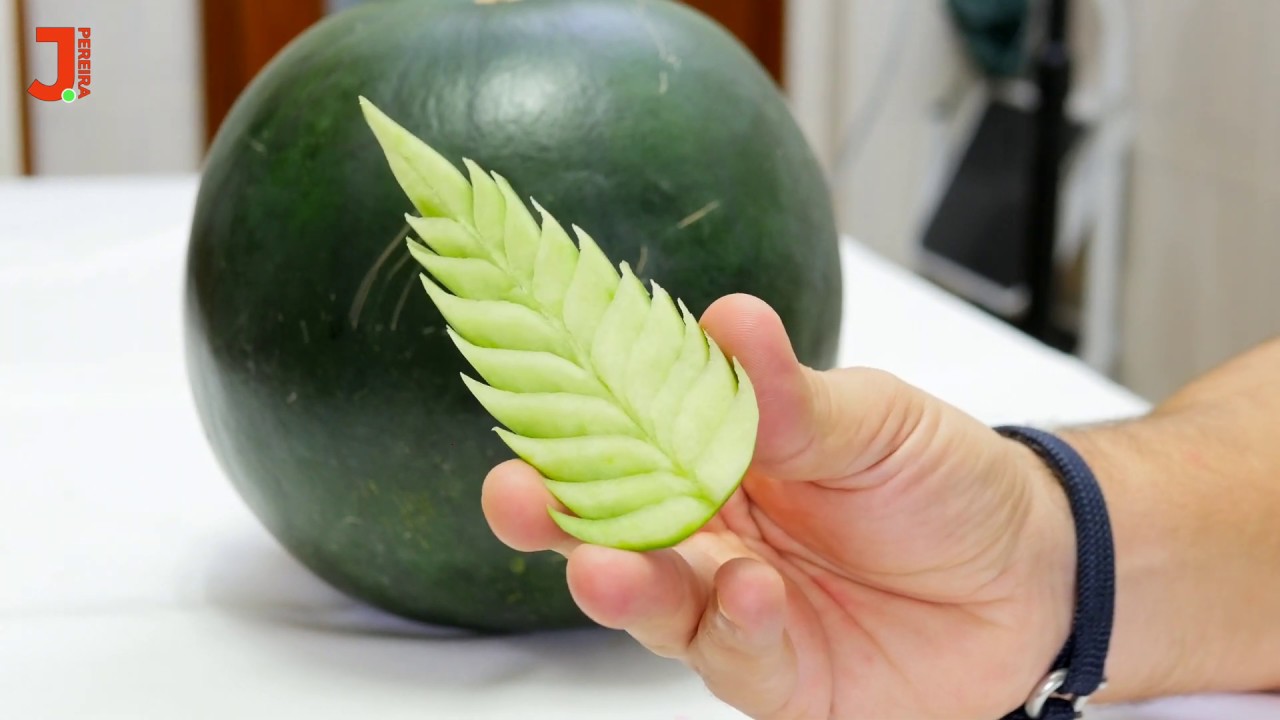The image displays a blurred background of what appears to be a room with white walls, a varnished brown door, and a white table. In the foreground, a pale Caucasian hand, with a slight amount of brown hair and wearing a blue-and-silver bracelet, is prominently holding a fruit or vegetable. This light green produce, possibly a honeydew or cucumber, has been intricately carved into the shape of a serrated dagger or arrowhead. It is being held between the thumb, index, and middle fingers of the person's right hand. Adjacent to the hand, on the white table, rests a large green ball that resembles either a watermelon or a bowling ball. In the upper left corner of the image, a red logo with a green leaf and text reading "Jay Pereira" can be seen clearly. The right side of the image shows a black-and-white object, though it's not entirely discernible due to the blur.